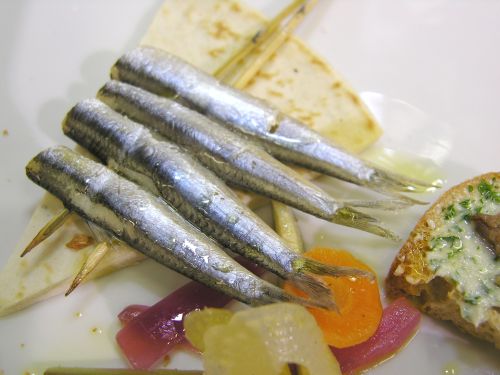The photograph depicts an up-close shot of a meticulously arranged food platter set on a solid white plate. Central to the image are four intact, headless sardines, skewered with wooden sticks and resting diagonally atop a triangular wedge of beige pita bread. Below the sardines, there is an assortment of sliced vegetables: a circular orange slice of carrot, a pinkish slice of pickled onion, and a yellow piece that could be ginger or another type of fruit. To the right of the sardines and vegetables, partially cut off at the corner of the image, is a thin piece of toasted crostini topped with melted cheese, a green herb, and possibly a small mushroom or another brown component. The lighting creates a soft reflection on the plate, adding to the detailed and appetizing presentation of the dish despite the sardines' rather unceremonious appearance with their heads removed.